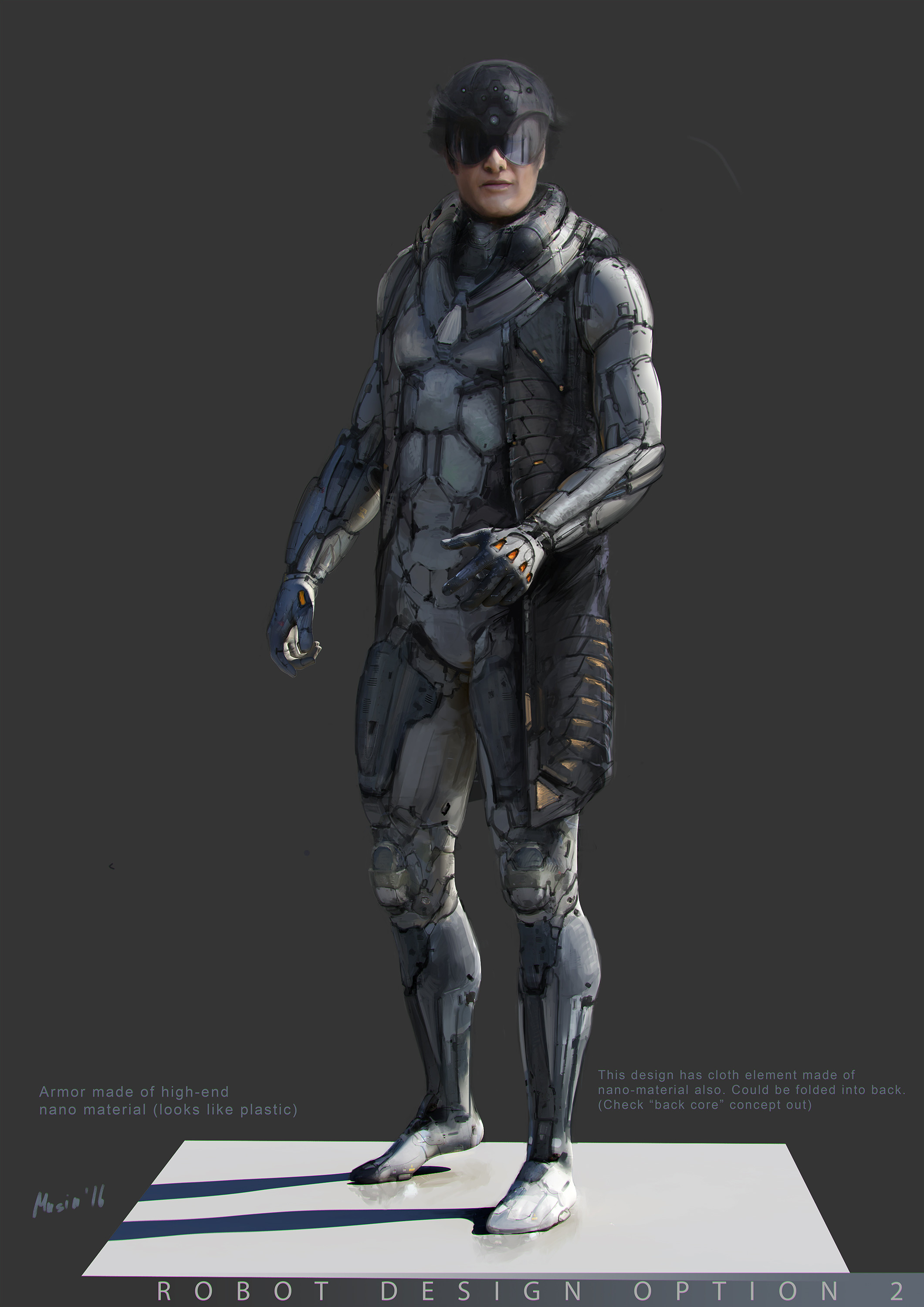The image showcases a detailed concept of a human-like robot standing on a white square platform against a deep gray background. The robot, which looks like it belongs to a graphic game or a design project, features an outfit that is predominantly dark gray and metallic, with segmented legs, arms, and chest giving it an artificial yet human shape. Notably, the head stands out with its human-like flesh tones and simple features, including a small triangular nose and mouth. It is adorned with a helmet and black ski-like goggles. The robot's left hand is reaching backward, while the right hand is open, palm facing forward, as if in a calming gesture. Beneath its feet, shadows stretch outwards, and there is tiny, faint text near its calves. The larger text at the very bottom of the image reads, "robot design option two." Additional notations inform that the robot's armor is made of high-end nanomaterial resembling plastic, and elements of its cloth can fold into the back, highlighting versatile design aspects.